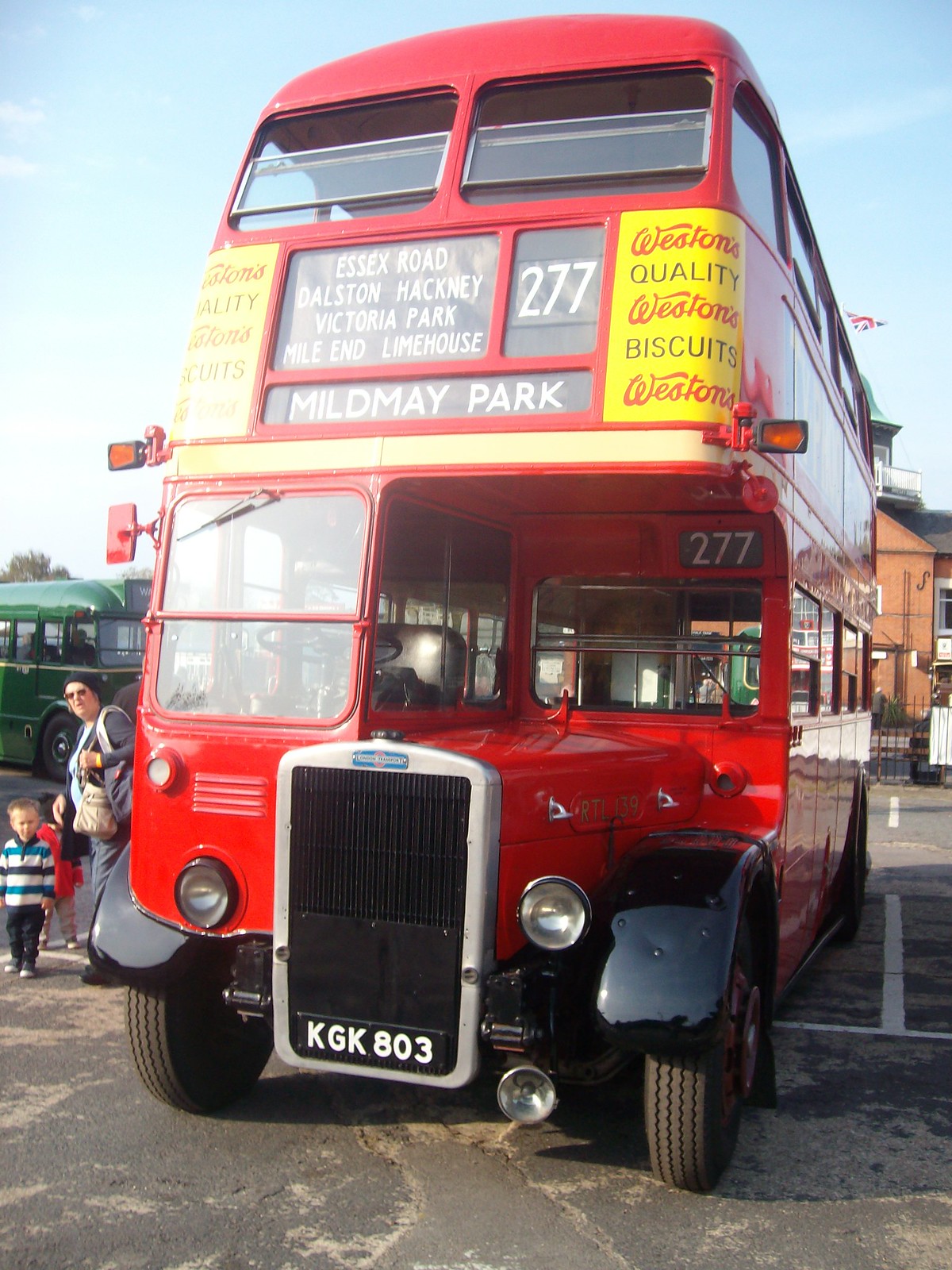This vertical rectangular photograph captures the front of a red, vintage, double-decker bus in a UK setting. The bus has both a bottom and an upper level, distinguished by various signs and advertisements. Prominently displayed on the front bumper is the license plate number, KGK803. The bus features advertisements on the upper deck that read "Westin's Quality" and "Westin's Biscuits" against a yellow background. Above the driver’s cabin, the bus is marked with the route number 277, with destinations listed to the left, including Essex Road, Dalston Hackney, Victoria Park, Mile End, and Limehouse. The bus stands on a worn, mixed gray street, with a clear blue sky adorned with a few white feathery clouds above. On the left side of the image, a woman and two children are seen observing the bus, reminiscent of onlookers or tourists. In the background, partially visible, is another bus with green sides and roof, along with a building that resembles residential housing.